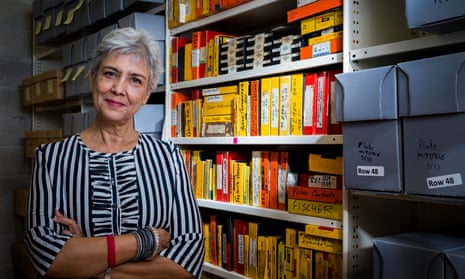This is a detailed photograph of an older Caucasian woman standing slightly to the left in what appears to be a file room. She is smiling subtly, with her lips turned upwards and adorned with pinkish-red lipstick. The woman has very short gray hair, styled close to the head. She is wearing a black and white striped blouse that features ruffles down the middle.

Her arms are crossed in front of her chest, and she is accessorized with a red bracelet on one hand and several other colorful beaded bracelets. The background reveals a large shelving unit filled with various items. The nearest shelf houses large white boxes labeled with black text and additional white labels. Further back, the central shelving section is cluttered with what appears to be numerous tapes or videos, identifiable by their red and orange hues and varied label directions. The furthest shelf holds smaller brown and white boxes, each marked with yellow post-it notes. The overall setting suggests a well-organized but densely packed filing system surrounding the woman.